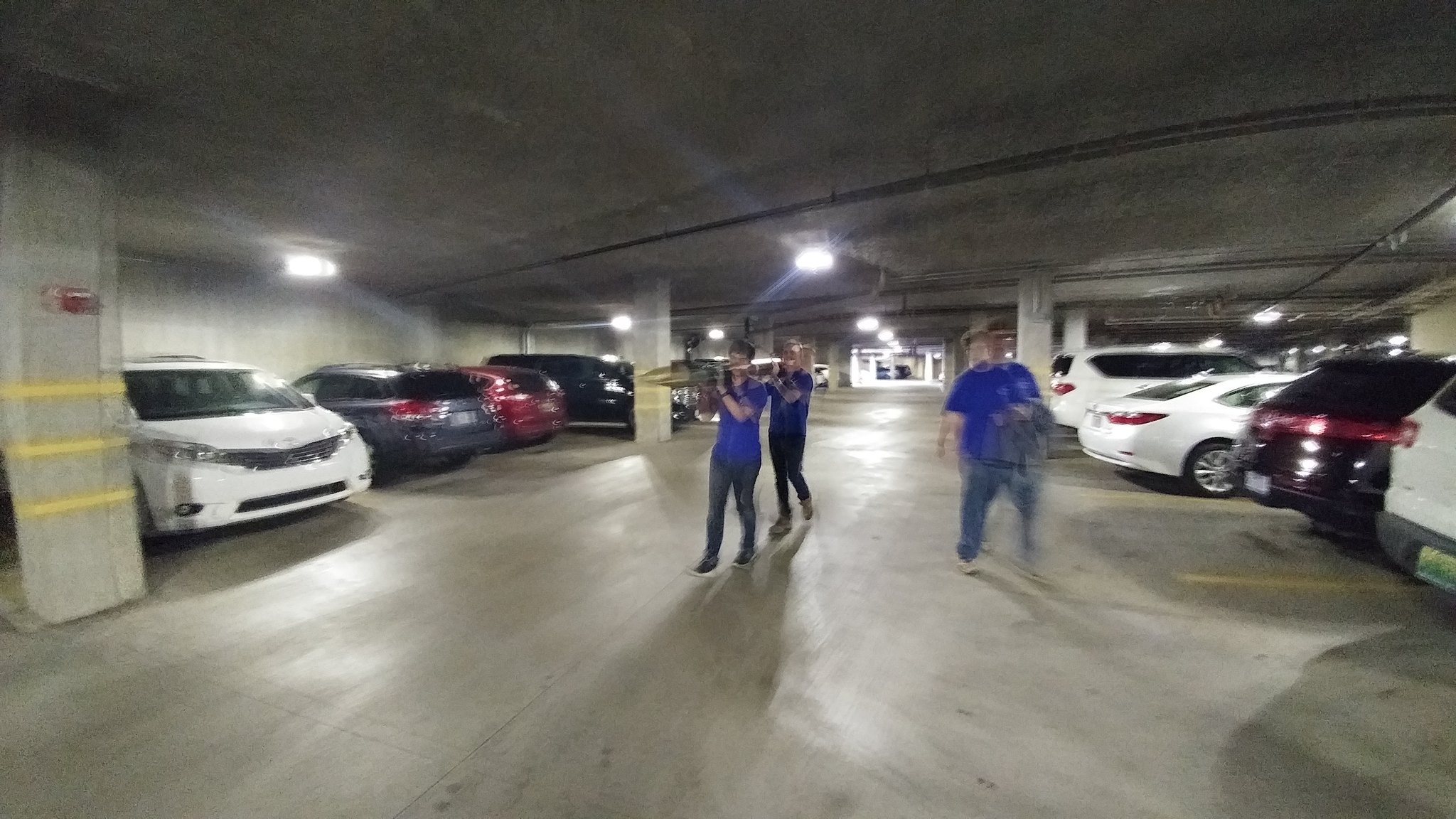This horizontal nighttime photograph captures an underground parking garage filled with a variety of vehicles occupying almost all the parking spaces. Most of the cars and trucks are parked head-in, except for a single van that is backed into its space. Positioned in the driving lane between two rows of parked cars, three young men are visible. Two of them are engaged in playing musical instruments, with the one in front playing a trombone. The third individual, standing to their right, is a larger figure holding a coat draped over his left arm. All three figures are dressed in matching blue t-shirts and dark trousers. Due to the motion and lighting conditions, the individuals and their activities appear slightly blurred, adding a dynamic and spontaneous feel to the scene.